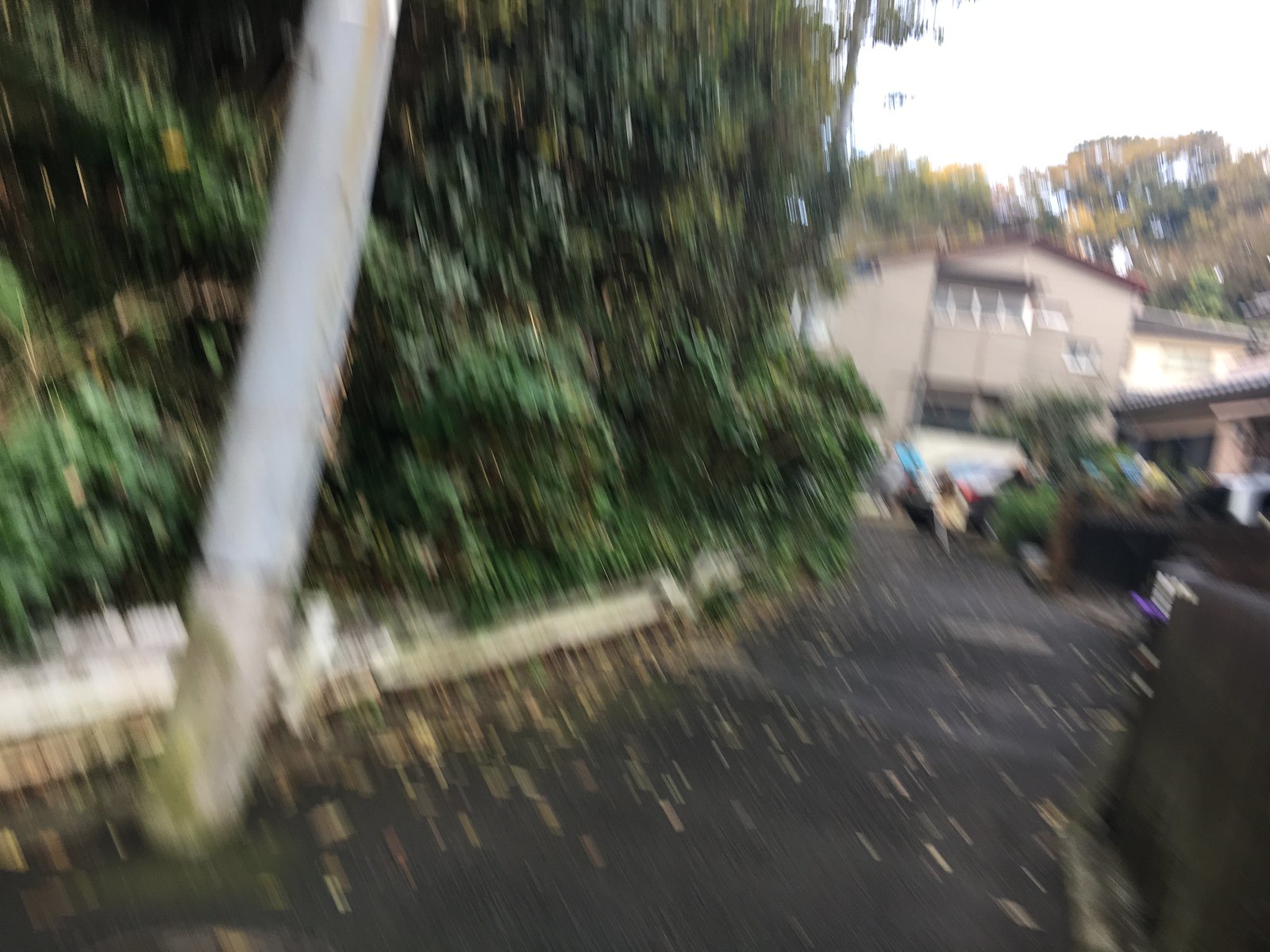The image depicts a somber yet intriguing scene of a two-story house with a recently renovated driveway. The driveway's foundation is a dark, fresh shade, indicating recent work. The house itself is built on a slight slope, giving it an uneven elevation that adds to its character. Along the left-hand side of the driveway, lush green trees provide a contrasting natural element to the otherwise stark scene. In front of the house, several cars are parked, and the area holds various unidentifiable items, adding an element of mystery to the overall composition.